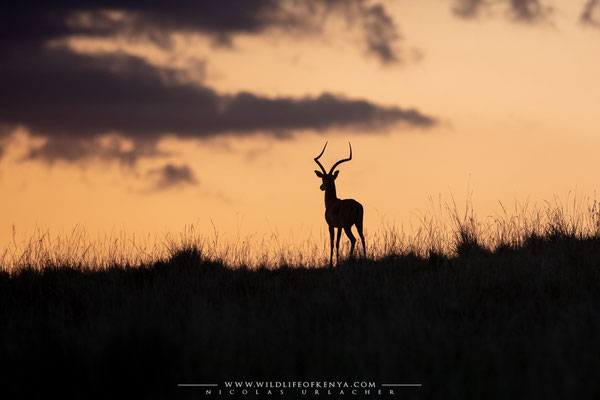This breathtaking color photograph was taken at dusk, just as the sun was setting. The sky displays a stunning palette of oranges, pinks, and light creams, providing a vivid backdrop tinged with dark, almost purple, clouds in the top left corner. The main subject of the image is a young buck, identifiable by his two antlers, standing in the middle of a grassy field. Both the buck and the grass are rendered in silhouette, appearing almost black against the illuminated sky behind them, giving a sense of tranquility and stillness to the scene. The antelope stands on what appears to be the side of a grassy hill, looking off into the distance, its form dark and shadowed. This evocative widescreen image is credited to www.wildlifeofkenya.com, Nicholas Urchelor.